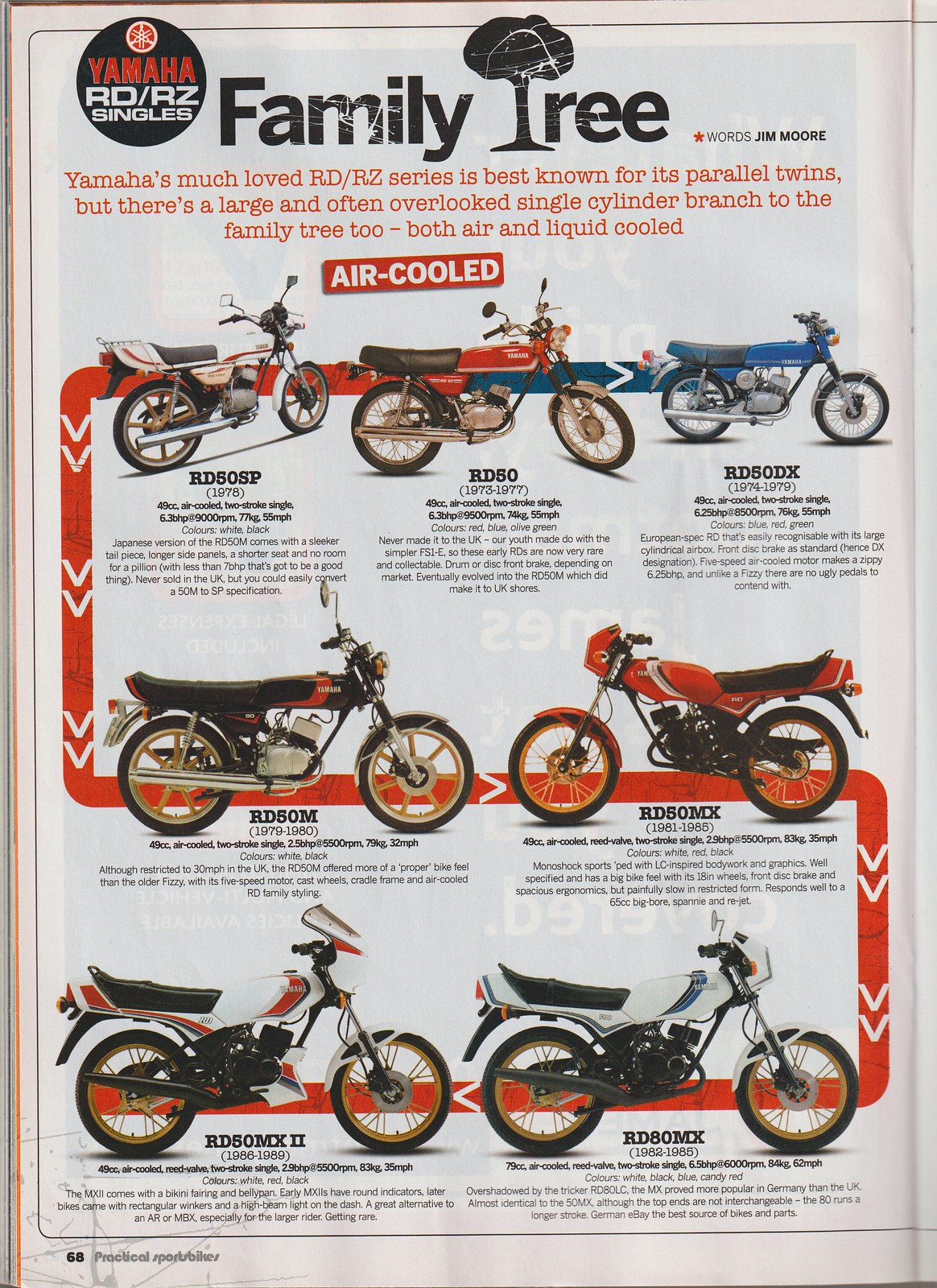This detailed magazine scan captures page 66 of Practical Sports Bikes, featuring an insightful exploration of the Yamaha RD-RZ singles family tree. The highlight of the page is the often overlooked single-cylinder branch of Yamaha’s RD-RZ series, famed primarily for their parallel twins. The focus here is exclusively on the air-cooled models, showcasing seven different motorcycles ranging from the 1970s to the late 1980s, with the most recent model appearing to be from 1989.

At the top of the page, the title "Yamaha RD-RZ Singles Family Tree" stands prominently, followed by the subtitle in striking red text: "Yamaha's much-loved RD-RZ series is best known for its parallel twins but there's a large and often overlooked single cylinder branch to the family tree too, both air and liquid cooled." The detailed descriptions of each bike are presented in black text.

Visually, the page is a vibrant collage of motorcycles in various colors – red, white, blue, and black – each distinctly upright and seemingly facing different directions, with two adjacent bikes facing each other. Although it remains unclear whether they are on kickstands, each model is meticulously displayed, harking back to an era of classic design and engineering. The specific models on display include the RD-50SP, RD-50, RD-50DX, RD-50M, RD-50MX, RD-50MX2, and RD-80MX. This visually engaging and informative layout serves as a nostalgic homage to Yamaha's enduring legacy of air-cooled, single-cylinder motorcycles.